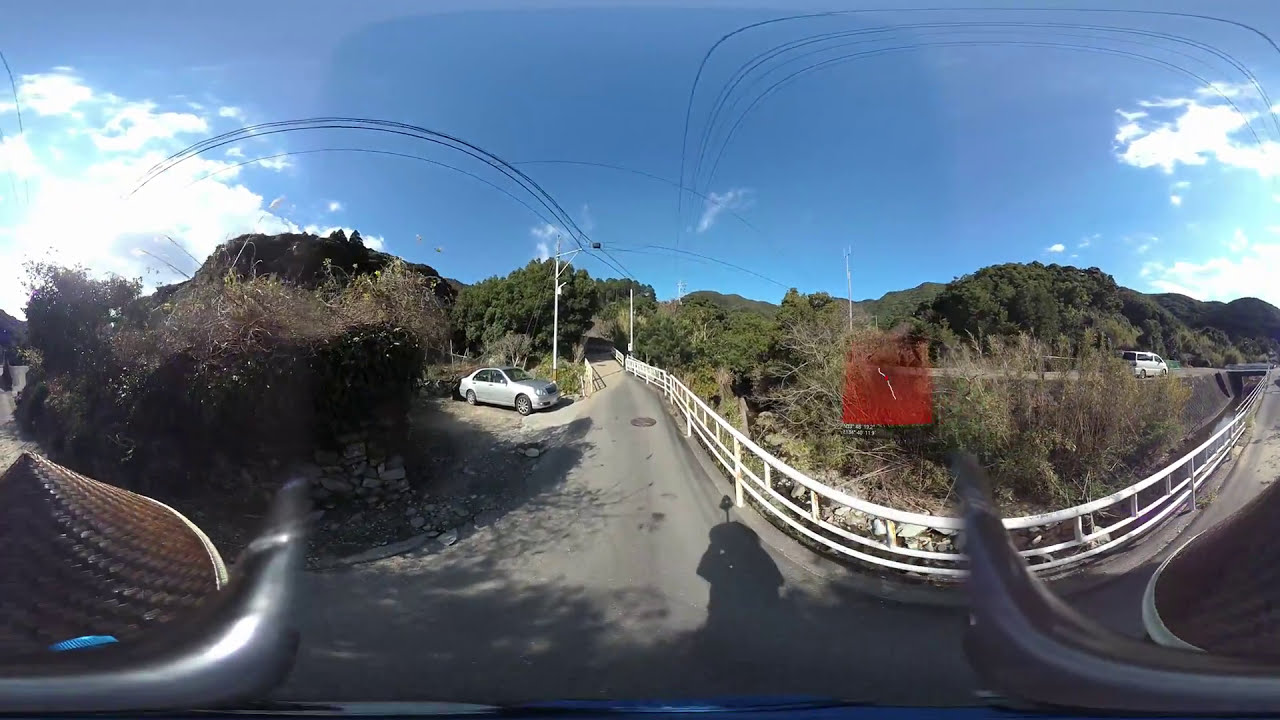The image captures a scenic outdoor area, likely a park or hiking spot, featuring a paved road or main street lined with white railings that extend along the sides. A single silver-gray car is backed into a parking spot off the main road, with a white van visible traveling in the distant right side of the image. The landscape is lush and green, adorned with numerous trees and bushes, along with a hillside or mountaintop covered in low-growing trees and sagebrush in the far background. Above, the sky is a bright blue with dispersed white clouds and wisps of black streaking through. Power lines hang overhead, and shadows from both the trees and photographer are evident, with the photographer's sun hat, made of brown, straw-like material with a pointed top, also visible. The overall setting is tranquil, blending natural and man-made elements harmoniously.